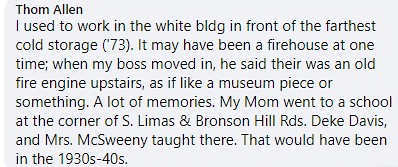The image features a block of black text on an opaque light gray background, formatted in a simple, sans-serif font. The text reads: "Tom Allen. I used to work in the white building in front of the farthest cold storage in 73. It may have been a firehouse at one time. When my boss moved in, he said there was an old fire engine upstairs, as if like a museum piece or something. A lot of memories. My mom went to a school at the corner of S. Lemus and Bronson Hill Roads. Deke Davis and Mrs. McSweeney taught there. That would have been in the 1930s to 40s." The entire image emphasizes a nostalgic reflection on personal and family history, possibly commenting on a photograph related to these memories.